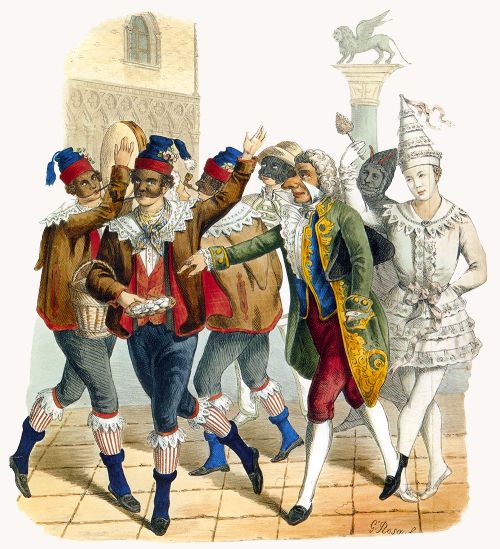The detailed illustration appears to be an elaborate, hand-colored etching, signed in script in the bottom right corner. It depicts a lively scene, possibly a masquerade ball happening outdoors in what looks like a medieval or 1700s court setting. The event features seven intricately-dressed figures who seem to be participating in a street performance or dance.

In the foreground, a central figure, likely a member of royalty, stands out with a distinctive appearance: a green coat trimmed with gold, a blue vest with gold embroidery, bright red pants, and black shoes. He wears a white powdered wig, a ruffled shirt, and has an exaggerated long nose. He is reaching out towards a group of entertainers. 

One entertainer, distinguished by an elaborate red, white, and blue hat, blue pants, and matching socks, is mid-dance, holding a tambourine. His attire includes striped red and white leggings and a basket draped across his arm. Another figure in similar clothing is depicted playing a drum overhead, while a third entertainer, also attired similarly, moves leftward and has his back to the viewer.

In the background, a tall column with a griffin statue on top stands prominently, showcasing the mythical creature with its wings raised. On the left side, partially obscured, is a brown building with a visible window. Other attendees include a figure dressed like a medieval knight and another person portraying a Pierrot clown, recognized by their white face paint, dunce hat, and short white dress with matching leggings and ballerina shoes.

The overall setting and attire suggest a festive, theatrical event, rich in historical costume detail and vibrant activity, capturing a vivid moment of aristocratic revelry and street entertainment.